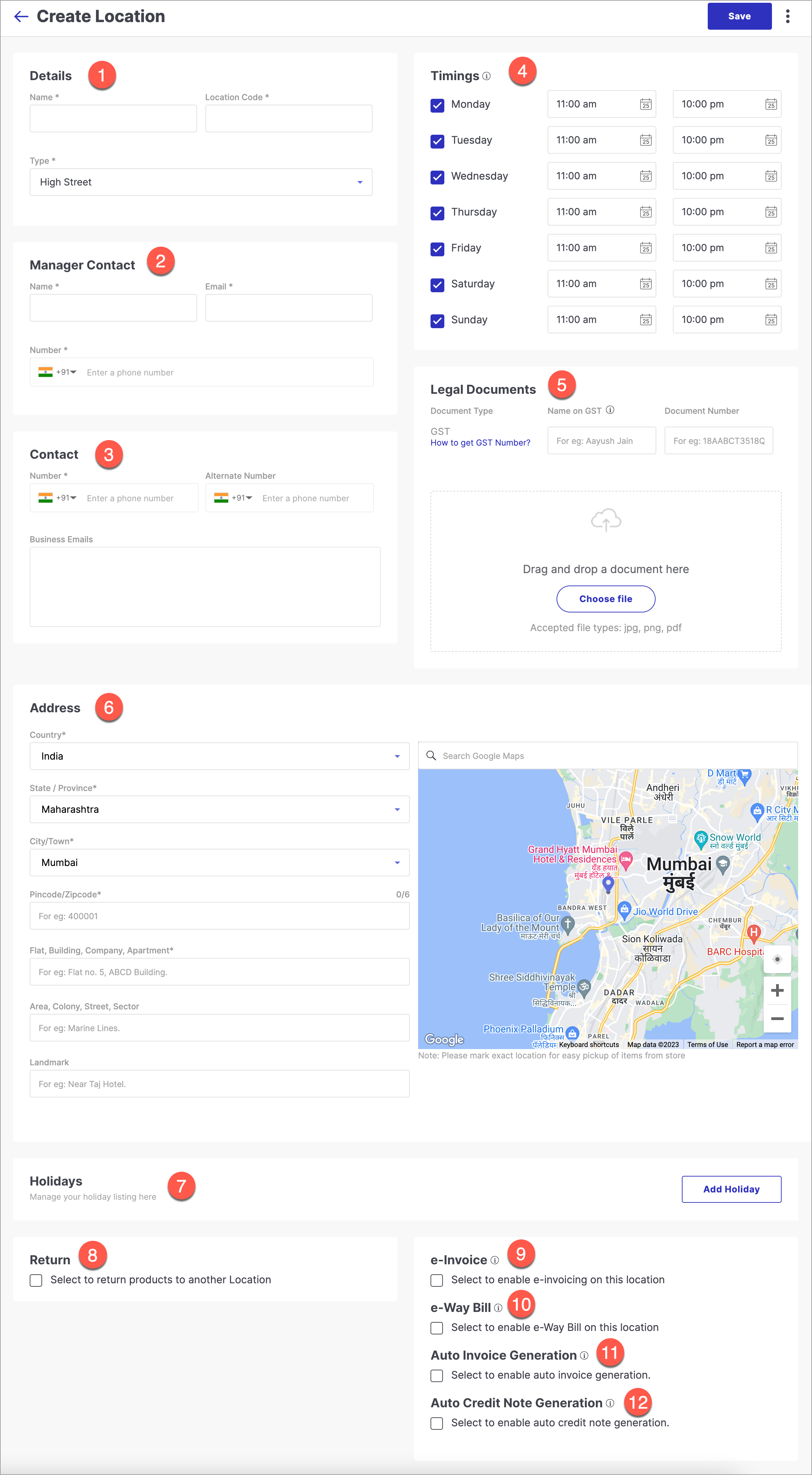The image depicts an informational form layout presented on a webpage, divided into square and rectangular sections with a clean white background. Each section is sequentially numbered and provides specific inputs and options. 

In the upper left-hand corner of the page, there is a label "Create Location." The upper right-hand corner features a "Save" button and a "More Options" button. Below this header, the form is organized into detailed, numbered sections. 

1. **Details**:
   - Boxes for "Name," "Location Code," and "Type" with a drop-down menu that selects "High Street."

2. **Manager Contact**:
   - Fields for "Name," "Email," and "Phone Number," accompanied by an Indian flag icon.

3. **Contact Numbers**:
   - Inputs for "Contact Number," "Alternative Number," and "Business Emails," also displaying the Indian flag icon.

4. **Timings**:
   - Days of the week (Monday to Sunday) each followed by blue check marks and the time "11 a.m. to 10 p.m."

5. **Legal Documents**:
   - Requires "Document Type," "Name on GST," and "Document Number."
   - A link titled "GST and how to get GST number" is clickable.
   - Includes a drag-and-drop feature for documents, and a "Choose File" option.

6. **Address**:
   - Detailed fields for "Country" (India), "State/Province" (Maharashtra), "City Name" (Mumbai), "Zip Code," "Flat/Building/Company/Apartment," "Area/Colony/Street/Sector," and "Landmark."
   - A Google Map next to the address fields.

7. **Holidays**:
   - Option to "Add a Holiday."

8. **Return**:
   - An option to "Select to return products to another location."
   
9. **E-Invoice**.

10. **E-Way Bill**.

11. **Auto Invoice Generation**.

12. **Auto Credit Note Generation**.